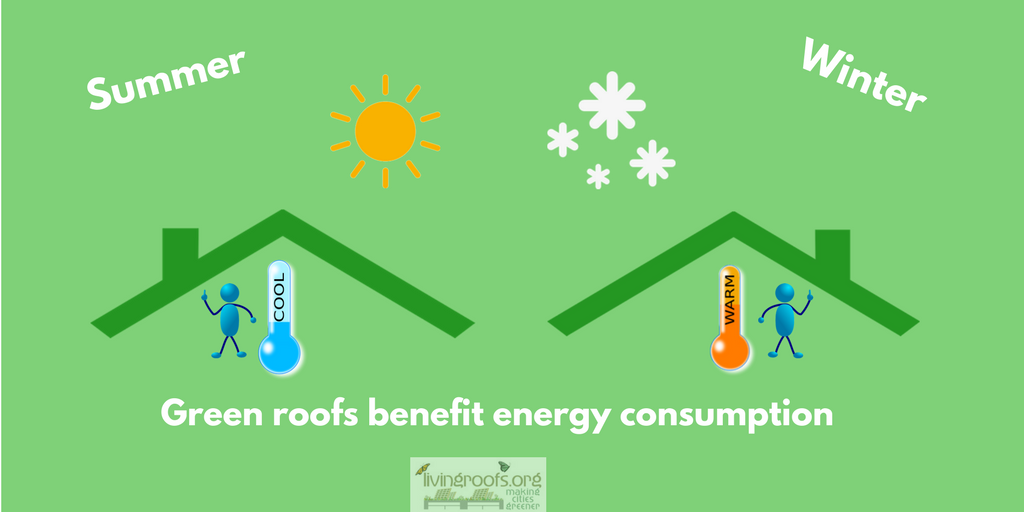The image is a digital illustration with a light green background and white text. In a diagonal on the top left, it declares "summer" accompanied by a simple yellow sun with radiating lines. On the left, there is a green outline of an arched roof with a rectangle representing a chimney. Below the roof, there's a blue stick figure with a rounded capsule body, round head, black arms, blue feet, and blue hands standing next to a blue thermometer labeled "cool.” 

On the right side of the illustration, the top corner reads "winter," also in white text. This side features a similar green roof outline with a chimney, beneath which is the same blue stick figure, now next to an orange thermometer marked "warm." Above the roof outline, various white asterisks symbolize snowflakes. 

At the bottom of the image, the text proclaims, "green roofs benefit energy consumption." Just below, there is a logo and text for livingroofs.org, slightly transparent, with the tagline, "making cities greener." 

The overall design is cartoon-like, with no detailed house outlines, emphasizing the benefits of energy-efficient roofing solutions.